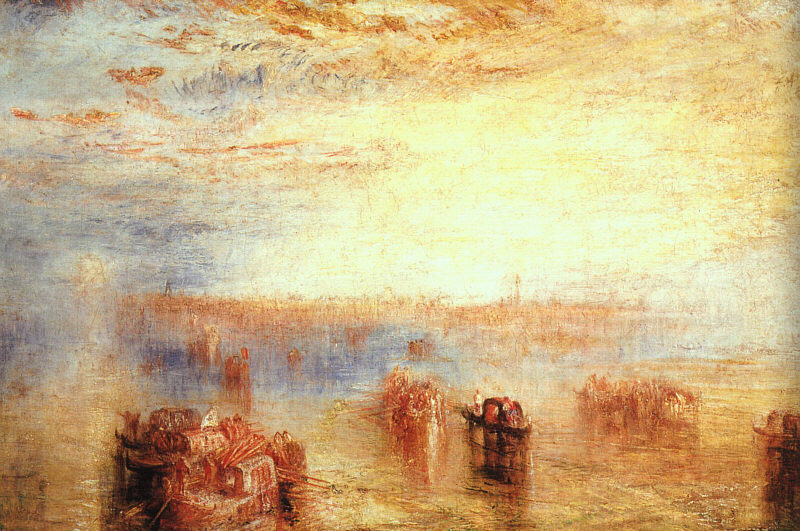This abstract painting features a water scene, predominantly using warm tones of gold, tan, and orange, with subtle blue accents. The sky and water blend seamlessly, making the horizon difficult to discern, with both the sky and water sharing similar light golden hues, sprinkled with darker brown tones. The scene appears to depict boats on water, with at least four discernible vessels that look heavily laden. Some boats have abstract figures, suggesting people, with one central boat seeming to carry multiple figures. The overall impression is one of movement, possibly symbolizing a journey, perhaps for freedom or a new life. In the background, there's a faint outline that could be interpreted as an island or tall brown grass, adding depth to the scene.